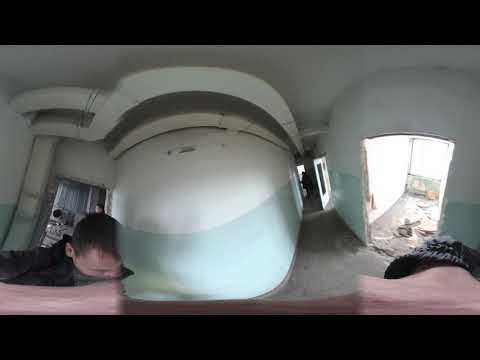This image, likely taken with a security camera or a VR 360 lens, shows a concrete room viewed from an elevated angle. The room's floor and walls are entirely concrete. In the center, there is a large, cylindrical structure, green on the bottom and white on top, resembling a living pod or storage tank. This central structure divides two hallways. On the right, there's an open doorway leading outside to a bright, sunlit area. Above, the ceiling features visible ducts and pipes. On the left side of the image, a person, possibly a white male with short hair wearing dark clothing and part of their face covered, can be seen looking down. This person appears again due to the VR imaging effect, giving a distorted, continuous view of the environment. The overall scene is slightly skewed, with black borders at the top and bottom of the image, suggesting an unusual lens was used.